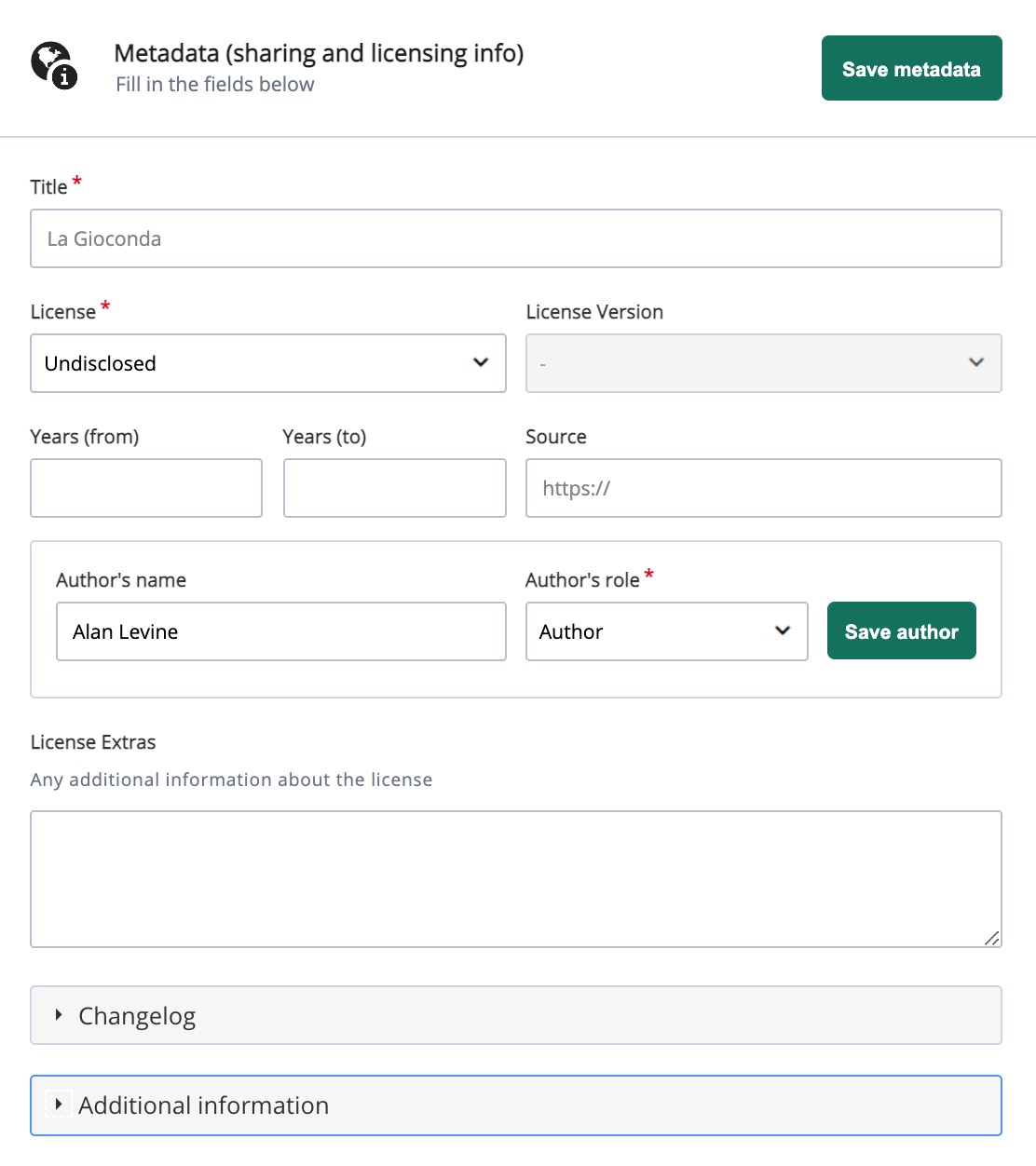The image depicts a metadata entry form specifically designed for sharing and licensing information related to books. This area allows authors and publishers to fill in details such as titles, licensing versions, publication years, and other pertinent author information. The form appears to be intended for platforms like Amazon, where books can be sold and managed. It provides a structured space to ensure all necessary metadata is accurately entered for proper cataloging and discovery.